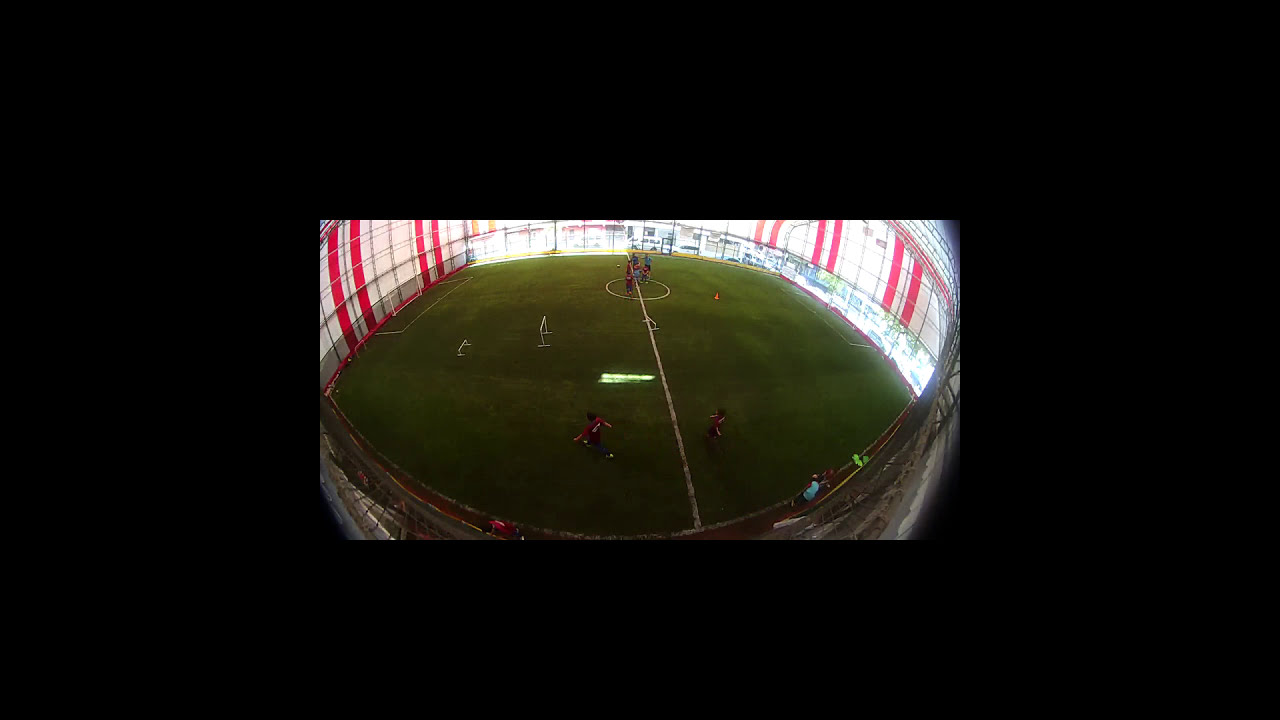The image depicts an indoor soccer complex captured from a high vantage point, potentially a mounted security camera or high-positioned photographer. The facility has tall, predominantly white walls adorned with vertical red stripes, creating a distinctive dome-like enclosure. The field, covered in vibrant green turf, features a clearly marked midfield line and goalposts at both ends. The lower section of the walls has numerous windows, allowing natural light to flood the space and providing outside views of a bright, sunny day with some trees visible. Players, dressed in maroon jerseys and black shorts, are engaged in various soccer drills rather than a full game. An orange pylon is positioned on the right side, where a few spectators are also present. The bright and partially open-air ambiance suggests a warm climate. The fisheye lens effect slightly distorts the image, emphasizing the circular shape of the field and the surrounding thick border that frames the view, giving an impression of a small, rectangular window through which this vibrant scene is observed.